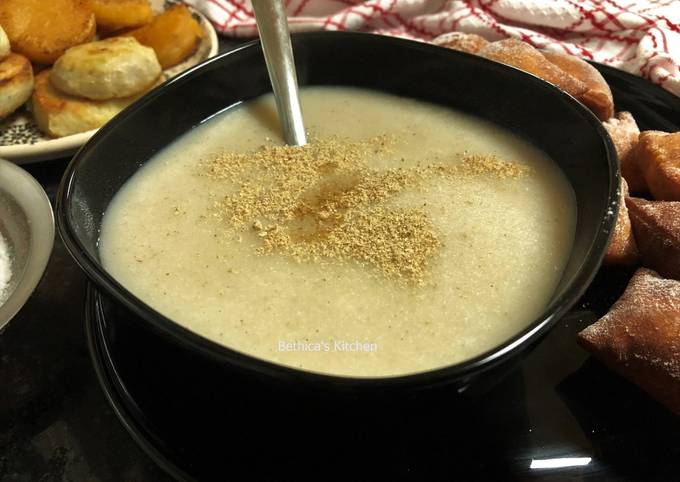This detailed close-up food photo captures a homely and hearty breakfast setting. Central to the image is a black bowl filled with what appears to be grits, sprinkled generously with brown sugar, and a spoon emerging from the bowl, suggesting it's ready to be enjoyed. The bowl rests on a matching black plate, creating a striking contrast against the off-white dish. Scattered on the same plate to the right of the bowl are dark brown sopapillas, lightly dusted with powdered sugar, adding a tempting touch. To the left of the bowl, a small silver dish with a wide edge contains a hint of additional powdered sugar, barely making it into the frame. Positioned near the top left corner, there's a white plate with blue accents holding a stack of fluffy, round biscuits, further enhancing the breakfast theme. Completing the cozy scene, a white kitchen towel with red stripes is draped in the background. Notably, in small text on top of the grits, are the words "Bethica's Kitchen," adding a personal and inviting touch to the meal.